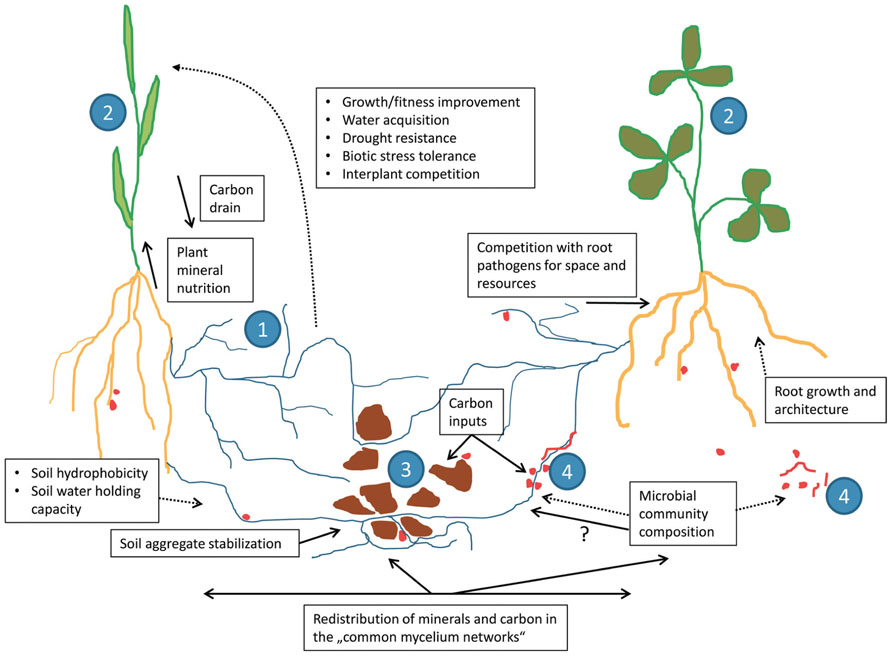This detailed infographic illustrates the mechanisms of plant root systems. It features two simply drawn green plants at the top, labeled with blue circled numbers. The roots extending below these plants are depicted in orange, with additional blue lines and brown rocks interspersed among the roots. Red dots further detail the intricate underground system. The diagram is rich with specific text boxes and captions, highlighting various aspects of the root functions and interactions, such as growth, fitness improvement, water acquisition, drought resistance, biotic stress tolerance, and interplant competition. Additional annotations describe more intricate processes: carbon drain, plant mineral nutrition, soil hydrophobicity, soil water holding capacity, soil aggregate stabilization, carbon inputs, competition with root pathogens for space and resources, root growth and architecture, and microbial community composition. At the base of the diagram, arrows and a label summarize the redistribution of minerals and carbon within the common mycelium networks, providing a comprehensive understanding of the interconnected plant-soil-microbial system. Overall, the infographic serves as a detailed and educational representation, suiting both scientific study and instructional use.